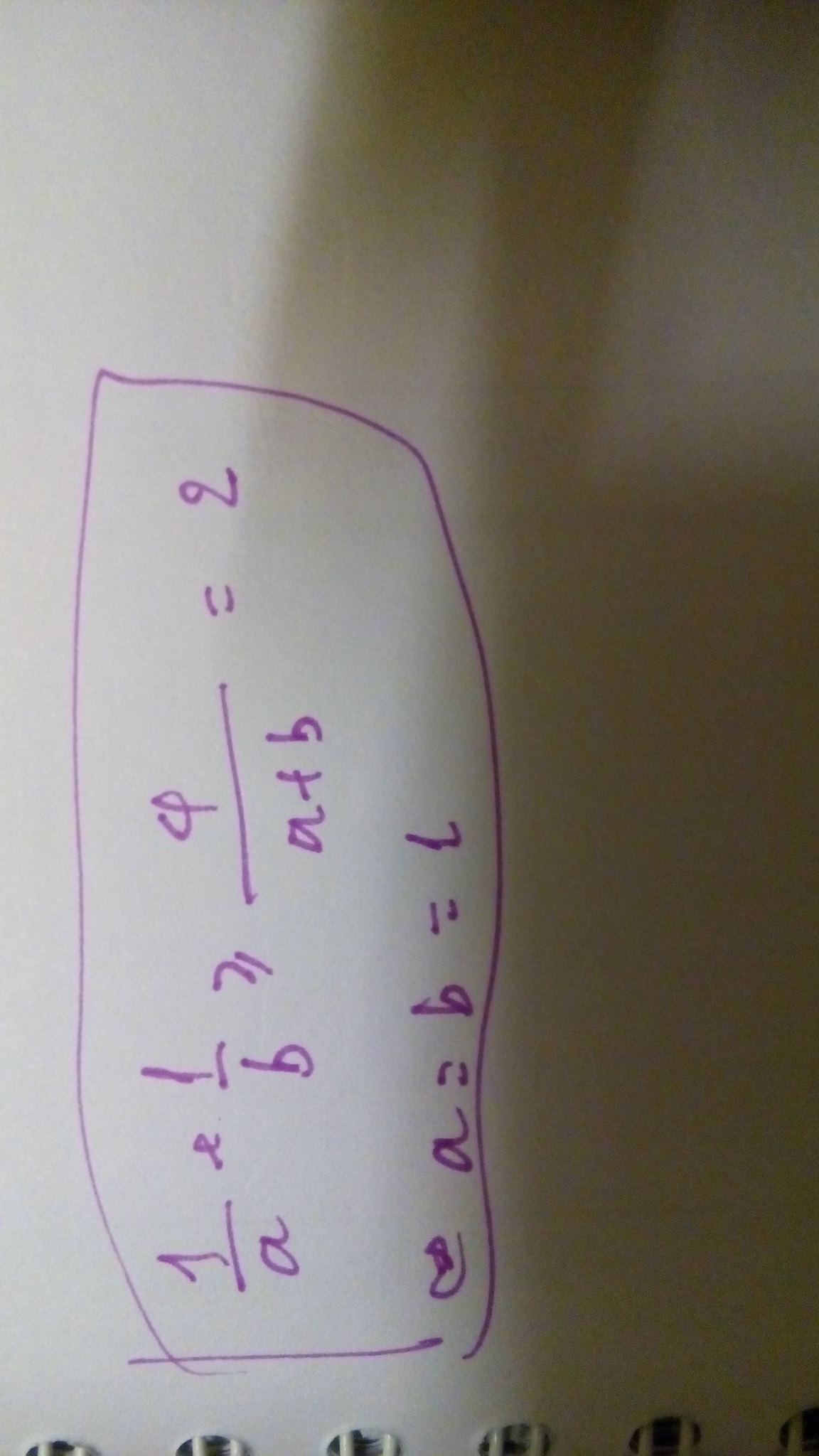This image is a close-up photograph of a piece of white notebook paper. Six double metal rings are visible at the bottom edge of the frame, indicating that the paper is part of a ring-bound notebook. The right side of the image is heavily shaded, casting a significant shadow over that portion. The writing on the paper, done in purple ink, is oriented 90 degrees to the left. The mathematical formula reads "1/A ⬨ 1/B ≥ φ/(A + B) = 2." Below this, another line of text in purple ink states "⬨ A = B = L." The entire set of equations is enclosed within a hand-drawn rectangular border, with the top (left side of the page) and bottom (right side of the page) lines being notably flatter. The image provides a detailed and intimate glimpse of the mathematical notations jotted down, with particular attention given to the shading and the notebook's metal rings.